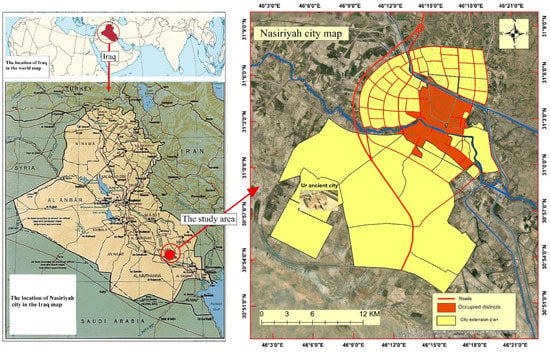The image features two distinct maps in color. On the left side, there is a map of Iraq, with a section at the top labeled "Iraq" and a box at the bottom highlighting the location of Naziriyah City. A red dot encircled with an arrow points across to the right map, marked as "the study area." This left map also includes small text indicating Iraq’s position globally relative to other countries.

The right map is a more detailed depiction of Naziriyah City, titled "Naziriyah City map" at the top. This map features a compass rose in the top right corner to display cardinal directions (north, west, east, south). The map itself is drawn predominantly in yellow and red, with a legend explaining that red signifies occupied districts and yellow signifies city areas. Additional elements include a small box marked “the ancient city” and a scale bar at the bottom showing distances of 0, 3, 6, and 12 kilometers. Blue lines indicating roads also crisscross the area.